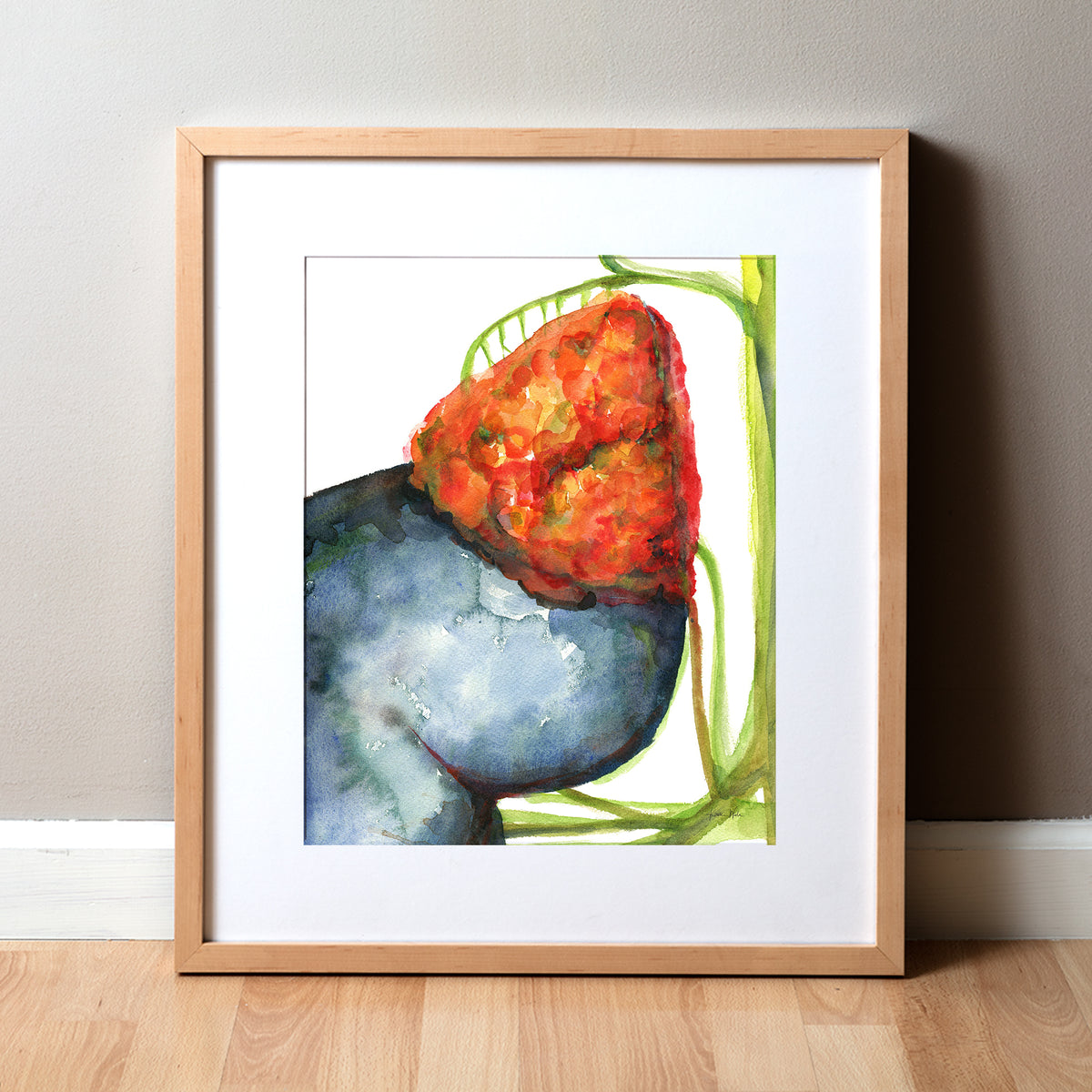This is a detailed color photograph featuring a painting within a light brown, possibly bamboo, frame. The painting is propped against a gray wall with white trim, on a light brown wooden or wood-like vinyl floor. Shadows are visible to the right of the frame. The art itself depicts a somewhat ambiguous subject that resembles a hybrid between a plant and an aquatic creature. Dominating the right side is a light green stem. Attached to it is a reddish shape reminiscent of an upside-down strawberry with hints of yellow and green, while the center features a triangular, gold-orangey head with bubble-like roundness, akin to a goldfish. Extending from this head, a bluish body with gray splotches adds a fluid, eel-like form, curling upwards. The background of the painting is white, contributing to the overall contrast and focus within the artwork.